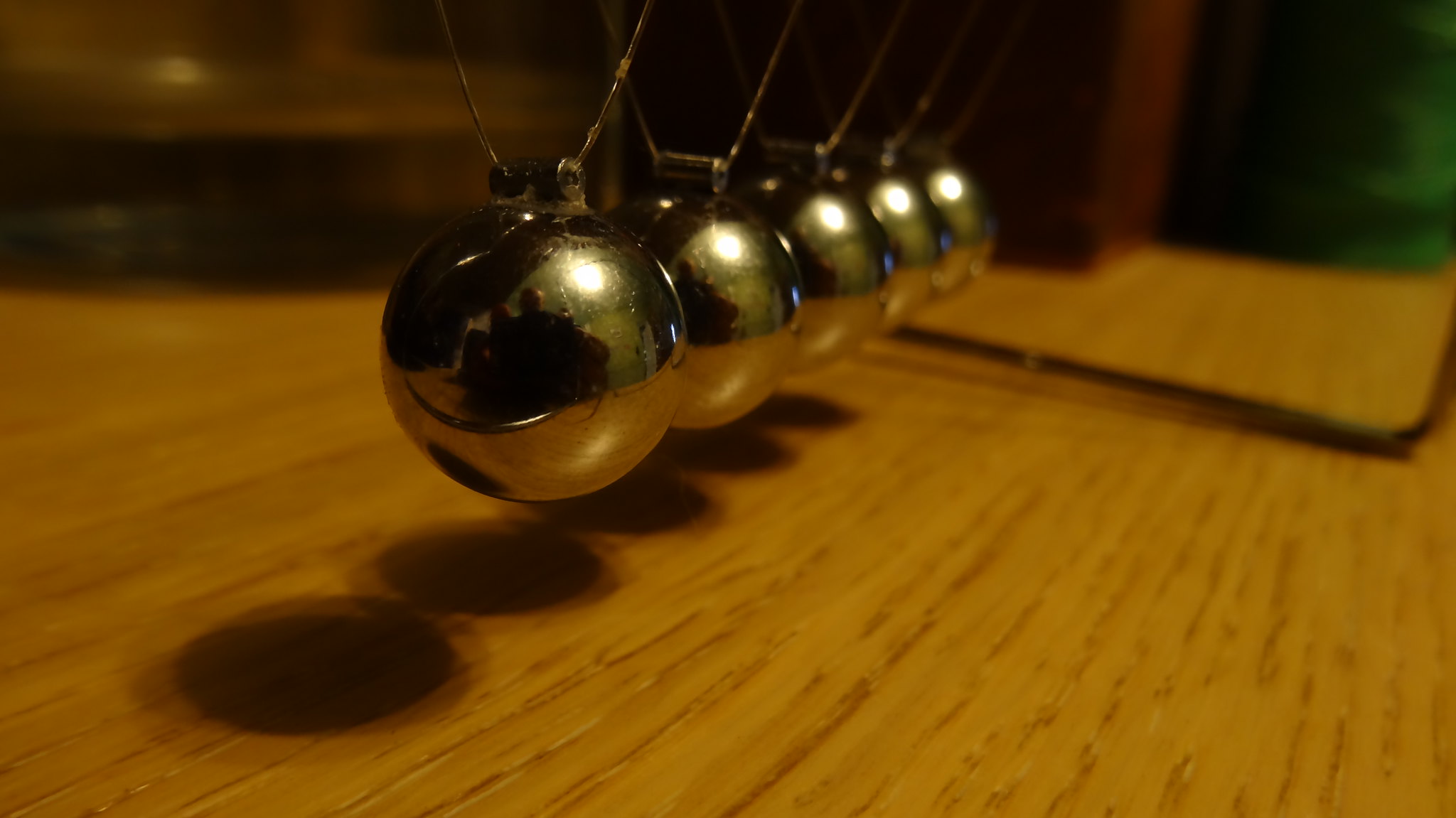This digital photograph captures a desk toy known as a Newton's cradle, featuring a black metal frame from which five gold balls are suspended by thin wires in a row. The balls, meant for demonstrating momentum and energy conservation, are about an inch above a light brown wooden surface with a fake wood grain design, featuring streaks of darker brown. The balls cast dark gray shadows directly beneath them, creating a noticeable contrast. The background of the image is blurry, with shades of brown transitioning to darker hues as one moves from left to right. The balls are positioned diagonally across the center of the landscape-oriented photo, and in the reflections of the first three balls, the silhouette of the photographer is faintly visible.